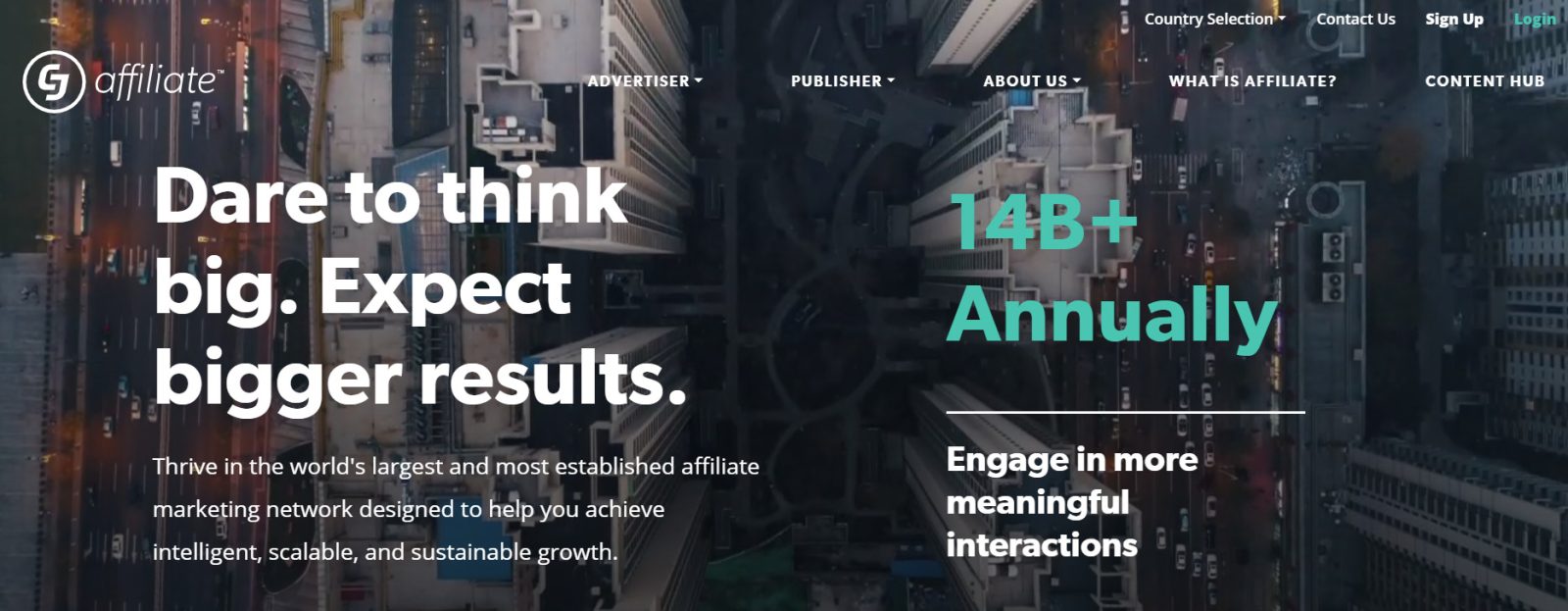This screenshot from the CJ Affiliate website highlights the core features and offerings of its affiliate marketing network. The interface prominently displays the CJ Affiliate logo at the top left, followed by a comprehensive navigation menu consisting of drop-down options for "Advertisers" and "Publishers," along with direct links to "About Us," an explanation of "What is Affiliate," a content hub, country selection, "Contact Us," "Sign Up," and "Log In." 

Anchoring the page, an aerial image of a bustling cityscape featuring high-rise buildings and busy streets serves as the dynamic background. At the forefront, a bold headline reads, "Dare to Think Big, Expect Bigger Results," with a compelling sub-headline stating, "Thrive in the world’s largest and most established affiliate marketing network designed to help you achieve intelligent, scalable, and sustainable growth."

A noteworthy statistic displays "14B+ annually," indicating the substantial annual engagements facilitated by the network, thereby cementing CJ Affiliate's position as a leader in the field. The emphasis on engaging in meaningful interactions further underscores the invitation for users to join the network, be they advertisers or publishers seeking scalable marketing solutions.

The design and layout not only showcase CJ Affiliate as a premier and large-scale network but also highlight the ease of navigation and action buttons to help users effortlessly access information and start leveraging the platform's capabilities. While the annual figure of 14 billion may seem ambitious, the overall presentation effectively promotes CJ Affiliate’s potential for fostering significant growth and interactions.